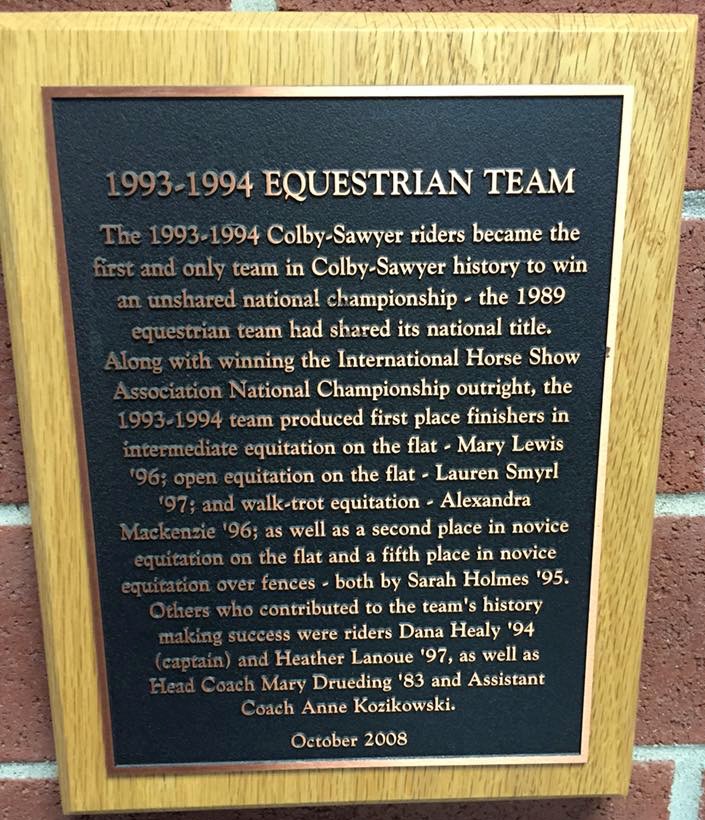The plaque, framed with a light yellowish wood border and mounted on a reddish brick wall, commemorates the 1993-1994 Colby-Sawyer equestrian team. The inscription highlights that the Colby-Sawyer Riders became the first and only team in the school's history to win an unshared national championship. It cites the 1989 equestrian team’s shared national title and victory in the International Horse Show Association National Championship. Detailing their achievements, the plaque lists first-place finishers Mary Lewis ’96 in intermediate equitation on the flat, Lauren Smurl ’97 in open equitation on the flat, and Alexandra McKenzie ’96 in walk-trot equitation. It also acknowledges Sarah Holmes ’95 for securing second place in novice equitation on the flat and fifth place in novice equitation over fences. The success is also attributed to riders Dana Healy ’94 (captain) and Heather Leno ’97, under the guidance of head coach Barry Druding ’83 and assistant coach Anne Koskowski. The text is elegantly displayed with a metallic sheen on a black background, complementing the plaque's distinguished appearance.